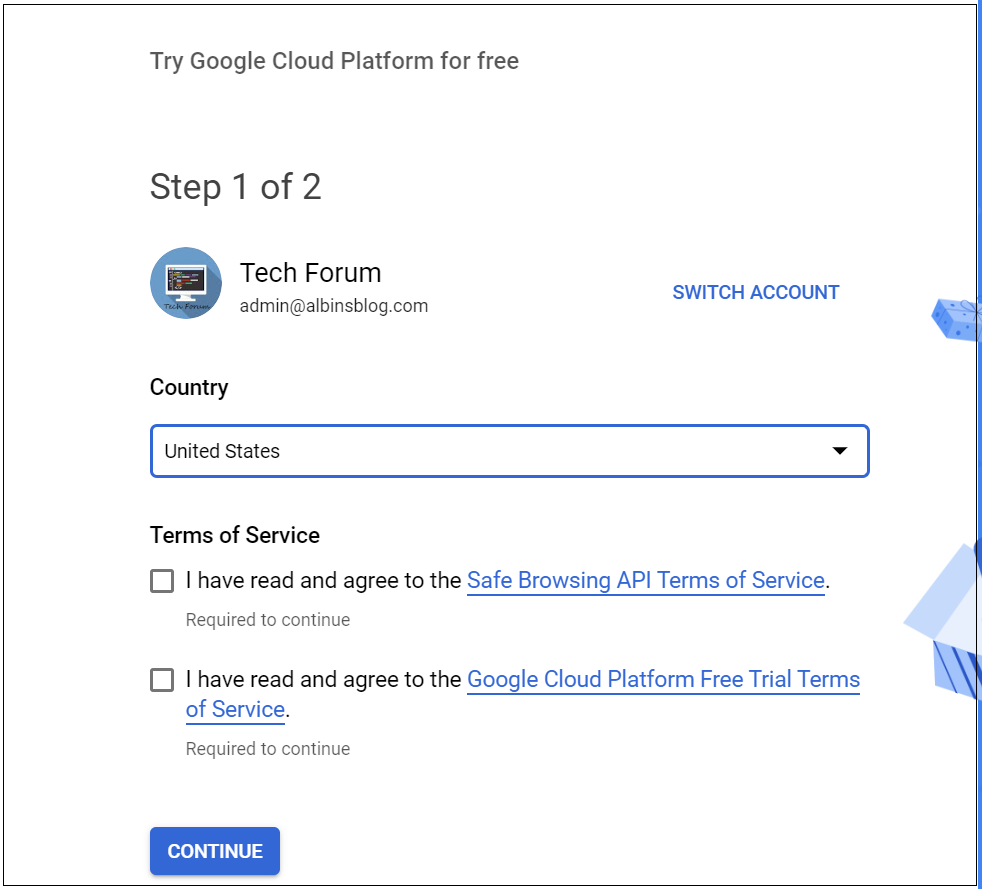**Caption for Google Cloud Platform Registration Page:**

This image captures the user interface of a registration page for the Google Cloud Platform (GCP) free trial, positioned under the category "Websites." The page is labeled "Step 1 of 2" and prominently features a blue circle with an icon of a computer monitor inside it. The user's status is identified as "Tech Forum Admin at albinsblog.com." In blue text, there's an option to "Switch account."

A country selection dropdown menu is displayed, with the "United States" currently selected. Below this, there are two checkbox options:

1. A statement declaring "I have read and agreed to the Safe Browsing API Terms of Service," which is clickable and required to continue.
2. A declaration stating "I have read and agreed to the Google Cloud Platform free trial Terms of Service," also clickable and required to continue.

Neither of these checkboxes are selected. Below these options is a prominently displayed blue button with white text that reads "Continue."

On the right-hand side of the page, there's a glimpse of a visually segmented box with light and dark blue stripes, potentially suggesting additional navigation or options. Above this segmented box, a small square with polka dots adds a decorative element to the page.